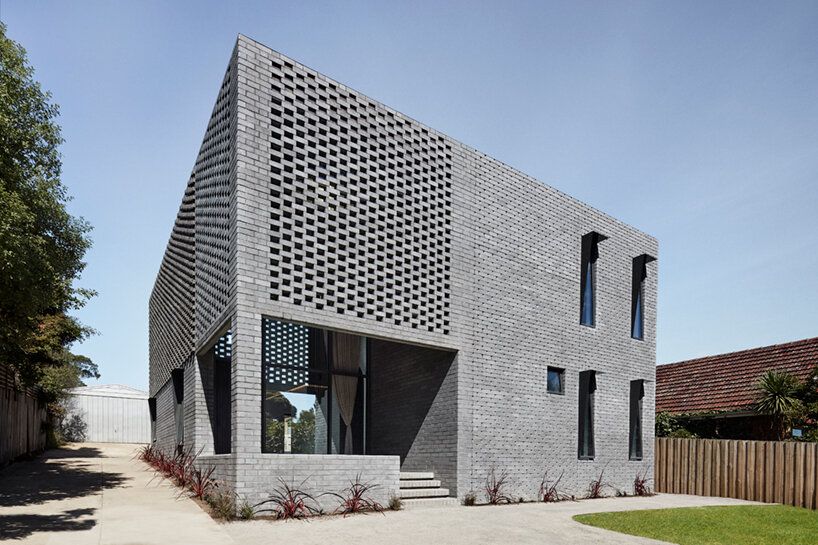The image depicts a sharp, modern-looking, two-story gray brick house with a flat roof, characterized by its clean, strong right angles and box-like rectangular shape. The front of the house is less wide than the sides, contributing to its distinct angular aesthetic. The brickwork is intricately designed, especially on the second-story front corner, where there's a brick column with a simple mortar stack, flanked by a creative pattern that resembles a basket weave, achieved by omitting every other brick.

The front facade features five windows—four being long and skinny, arranged vertically, with one small square window. These windows are defined by their black shutters, adding contrast to the gray brickwork. Below these windows, there's a gray-beige set of steps leading to an entrance porch. The entrance has large glass panels framed in black, and behind them, brown curtains are visible.

Minimal landscaping surrounds the house, including tiny shrubs with green and dark red leaves. The driveway and sidewalk are poured concrete, and a small yard with neatly cut green grass is present. A white panel fence encloses part of the property, with green-leaf trees interspersed. Additionally, a gray structure, likely a garage, can be seen towards the back. Another building with a brownish-red roof is visible to the right of the house, though the main focus remains on the detailed brick house with its modern architectural elements.